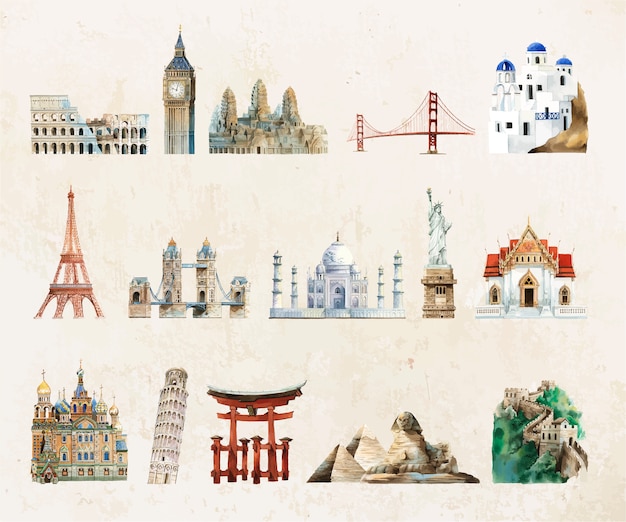This is a detailed illustration of 15 famous landmarks from around the world, depicted on a yellowish paper background. In the top row, from left to right, are the Colosseum, Big Ben, the Golden Gate Bridge, and a set of iconic white buildings with bright blue spired domes characteristic of Greek architecture. The second row features the Eiffel Tower, a notable bridge that might be the Tower Bridge of London, the Taj Mahal, the Statue of Liberty, and a temple-like structure with white walls and a red roof. The bottom row starts with a colorful building that could be a mosque or an Orthodox church with distinctive spires, followed by the Leaning Tower of Pisa, a shrine gate from Japan, the pyramids and the Sphinx at Giza, and finally, the Great Wall of China. This collection showcases architectural marvels from both the ancient and modern worlds.